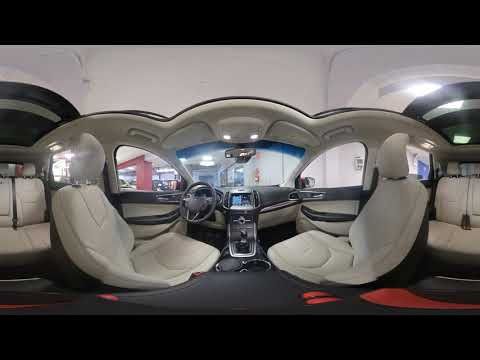This digital panoramic photograph captures the interior of a unique transport vehicle, viewed from the perspective of sitting inside. The image showcases various objects such as the steering wheel, gear shaft, console, mirrors, and radio, all clearly visible. Prominently featured in the center are two reclining style car seats directly facing each other. Surrounding these seats are additional upholstered seating areas: a bench style seat to the right of the console and other seats against the left wall. The vehicle's front and side windows offer a view of the exterior, revealing a parking garage or car dealership setting, with multiple buildings visible outside. The solid black border frames the image, enhancing the contrast against the vehicle's interior and the outdoor scenery. The photograph lacks any textual elements and features a color palette that includes black, gray, white, red, blue, tan, light green, beige, and yellow. This outdoor daytime scene provides a comprehensive view of this evidently high-tech vehicle inside its dealership environment.